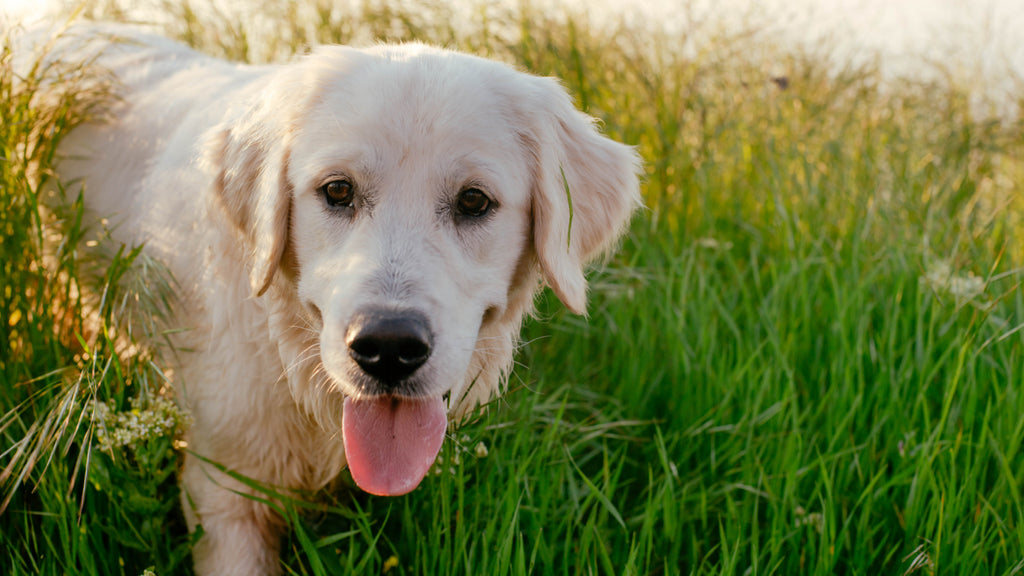In this photograph, a light off-white-yellow dog, likely a yellow lab, is captured mid-motion as it emerges from tall, green to golden-yellow-brown grass, its fur blending harmoniously with the natural hues of its surroundings. The landscape-oriented image places the dog on the left side, and it's apparent that the dog has been actively enjoying its time outdoors, evidenced by its pink tongue hanging out and a piece of grass adorning its ear. The dog, with its black nose and expressive dark brown eyes, gazes to the left, hinting at its playful and curious nature. Only the dog’s head, torso, and part of its front paws are visible, as the photograph is taken at the dog's eye level, giving a sense of intimacy and immediacy. A few delicate white flowers are scattered in the foreground, and the sky or distant landscape creates a pale backdrop in the top right corner. The setting feels like a meadow, with taller grasses and plants behind the dog and an insect captured in flight among the bushes to the right, adding a lively touch to the scene.